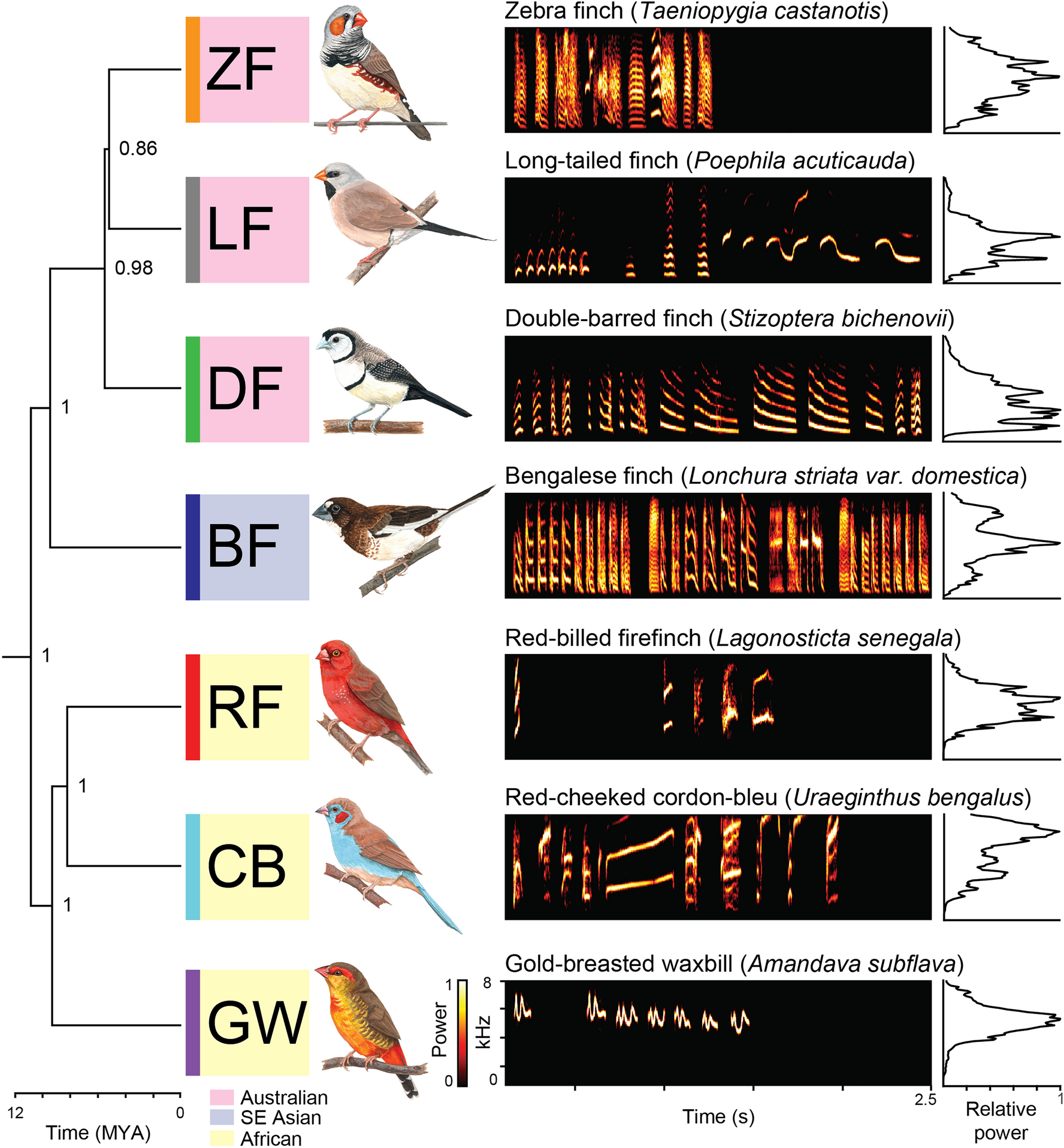The image features a detailed chart illustrating the songs of seven different bird species. Each row showcases an illustration of a bird alongside its initials, with identifiable drawings for the zebra finch (ZF), long-tailed finch (LTF), double-barreled finch (DBF), Bengalese finch (BF), red-billed fire finch (RBFF), red-cheeked cordon bleu (RCCB), and gold-breasted waxbill (GBW). Next to the bird illustrations, their scientific names are listed. To the right, each bird's song is visually represented through audiographs displaying the volume and duration of their chirps, with corresponding graphs indicating 'power' and 'time.' A legend explains the regional origins of the birds through color-coded blocks: pink for Australian, blue for Southeast Asian, and yellow for African, highlighting the geographical diversity of the species examined.